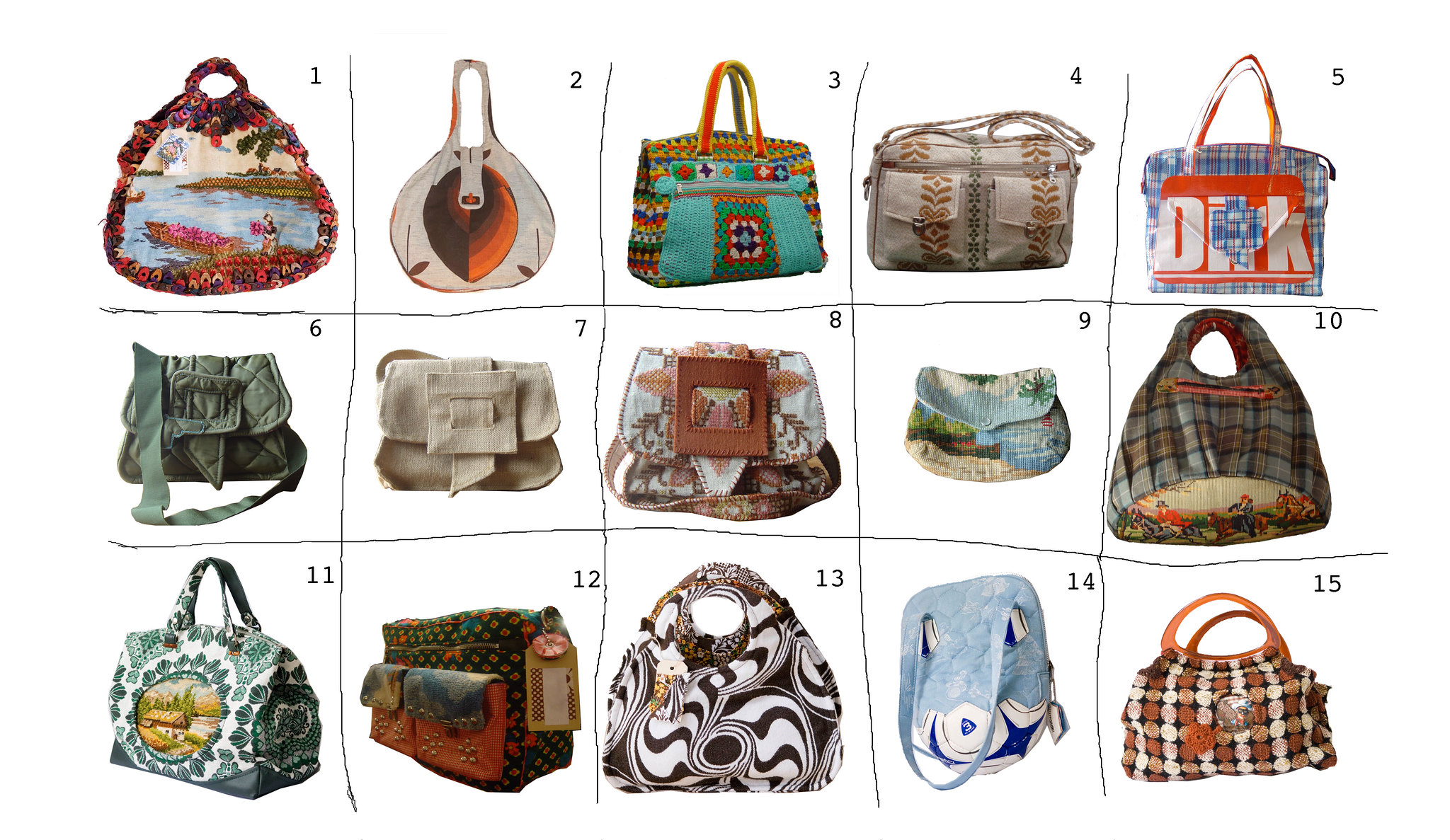In the image, a grid layout displays 15 distinct purses or bags, each positioned within its own numbered box, from 1 to 15. The black lines separating each box stand out against a white background. 

- The **top left bag**, numbered **1**, features a vibrant floral design with a handle.
- **2** is adorned with white and orange tones, sporting a large leaf shape in the center and has a handle.
- **3** boasts a crochet pattern in blue, orange, and yellow hues.
- **4** is embroidered with a brown leaf pattern on an ivory background.
- **5**, marked in an orange square with white font reading "OKK," showcases a blue and red plaid.

In the **second row**:
- **6** presents a quilted green pattern with various shades.
- **7** is designed with linen ivory and a prominent large buckle.
- **8** uses brown leather, featuring a detailed embroidered background in brown, white, and orange.
- **9** is a small, fold-over clutch depicting a tranquil blue water scene.
- **10** shows a plaid gray and red design with a depiction of people on horses at the bottom.

On the **bottom row**:
- **11** carries a white and green pattern, highlighting an outdoor barn scene in a circular frame.
- **12** integrates brown, red, and black patterns.
- **13** stands out with a mesmerizing swirly black and white design.
- **14** is a blend of subtle blue and white shades.
- **15** is dotted with a playful mix of brown, orange, and white circles, complete with an orange handle.

Each bag in this collage is uniquely vibrant, capturing a mix of patterns and textures, ranging from floral embroidery to plaid and swirly patterns, with a variety of shapes and color palettes, emphasizing the diversity in design.